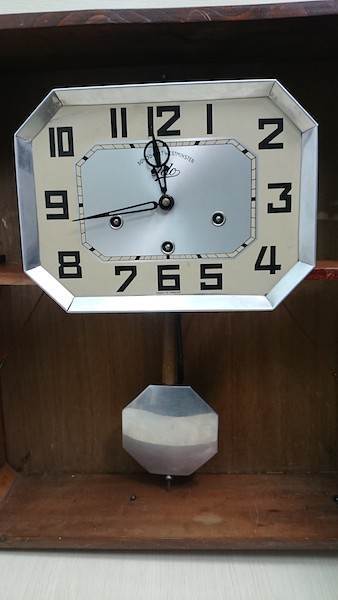This image depicts a silver-framed clock with an asymmetrical octagonal shape, housed within a medium to dark brown wooden cabinet. The clock face displays numerals from 1 to 12, unevenly spaced, with 11, 12, and 1 clustered closely together, as well as 5, 6, and 7. The clock shows the time as approximately 11:42 or 11:43. Positioned below the clock is a silver pendulum within a smaller, evenly shaped hexagon. The entire setup resembles a grandfather clock, set against a light gray or off-white background, and includes an insignia on the clock face that is unreadable.